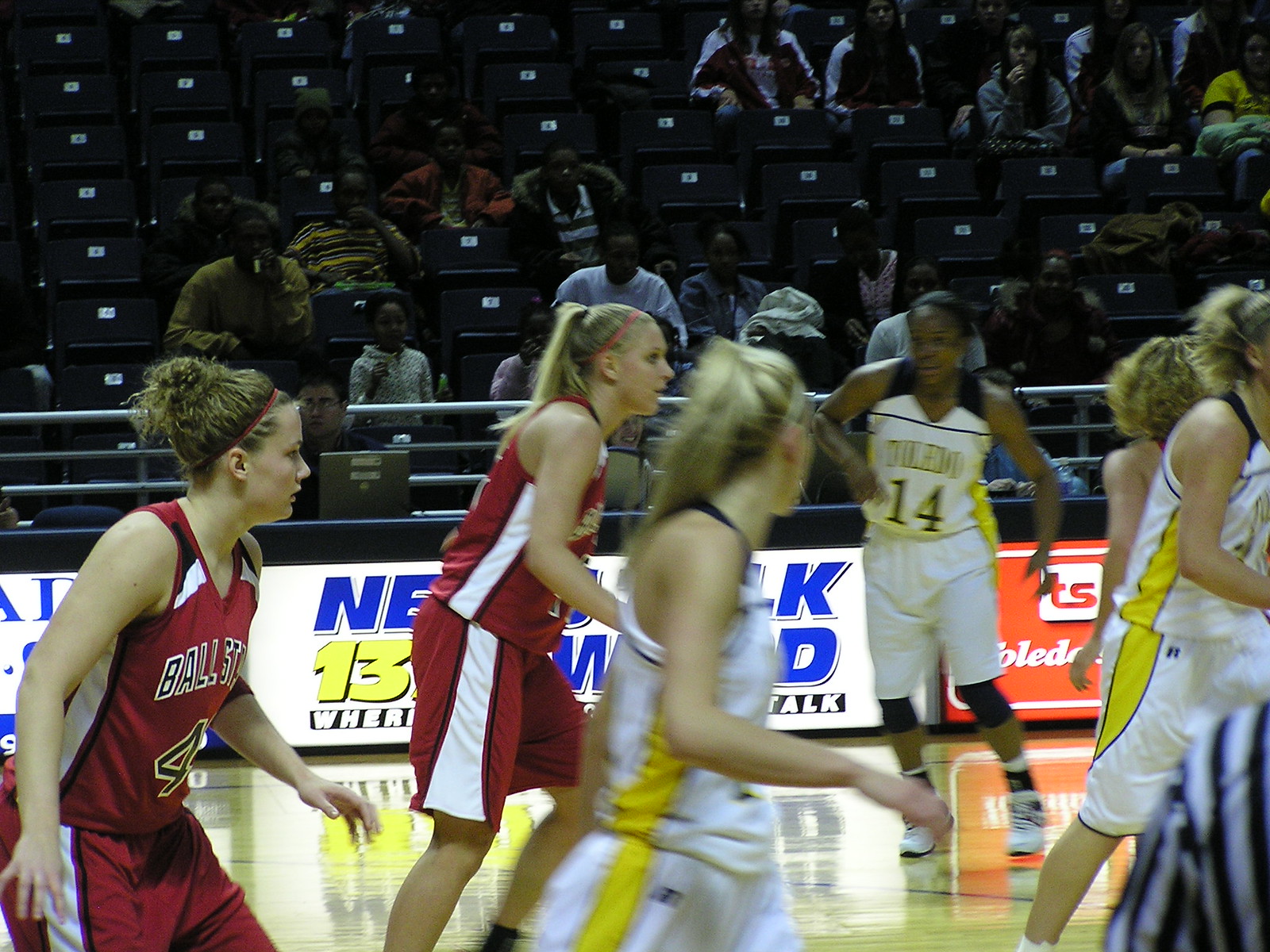The photograph captures an intense moment from a college women's basketball game on a well-lit indoor court. The image features six female players, divided into two teams. One team is dressed in red uniforms with white stripes, prominently displaying "Ball State" on their attire. Notably, player number 4 of this team has her hair pulled up in a ponytail secured with a headband.

The opposing team sports distinctive white uniforms with yellow stripes and black accents near the shoulders, identified as "Toledo." A focal point is player number 14, an African-American woman, while her teammates, all with blonde hair, focus on her attentively. One player closest to the camera has her blonde hair also tied back in a ponytail.

In the background, the sparse audience is seated behind metal railings, filling about a third of the available seats. Among the spectators, families with children can be seen. Signage around the court displays various, partially obscured, advertisements, including a red box with letters "TS" and blue lettering containing "L" and "K." An official referee, identifiable by their black and white striped shirt, is barely visible at the edge of the scene. The players on the court are in a ready stance, poised for continued action despite the basketball being out of frame.